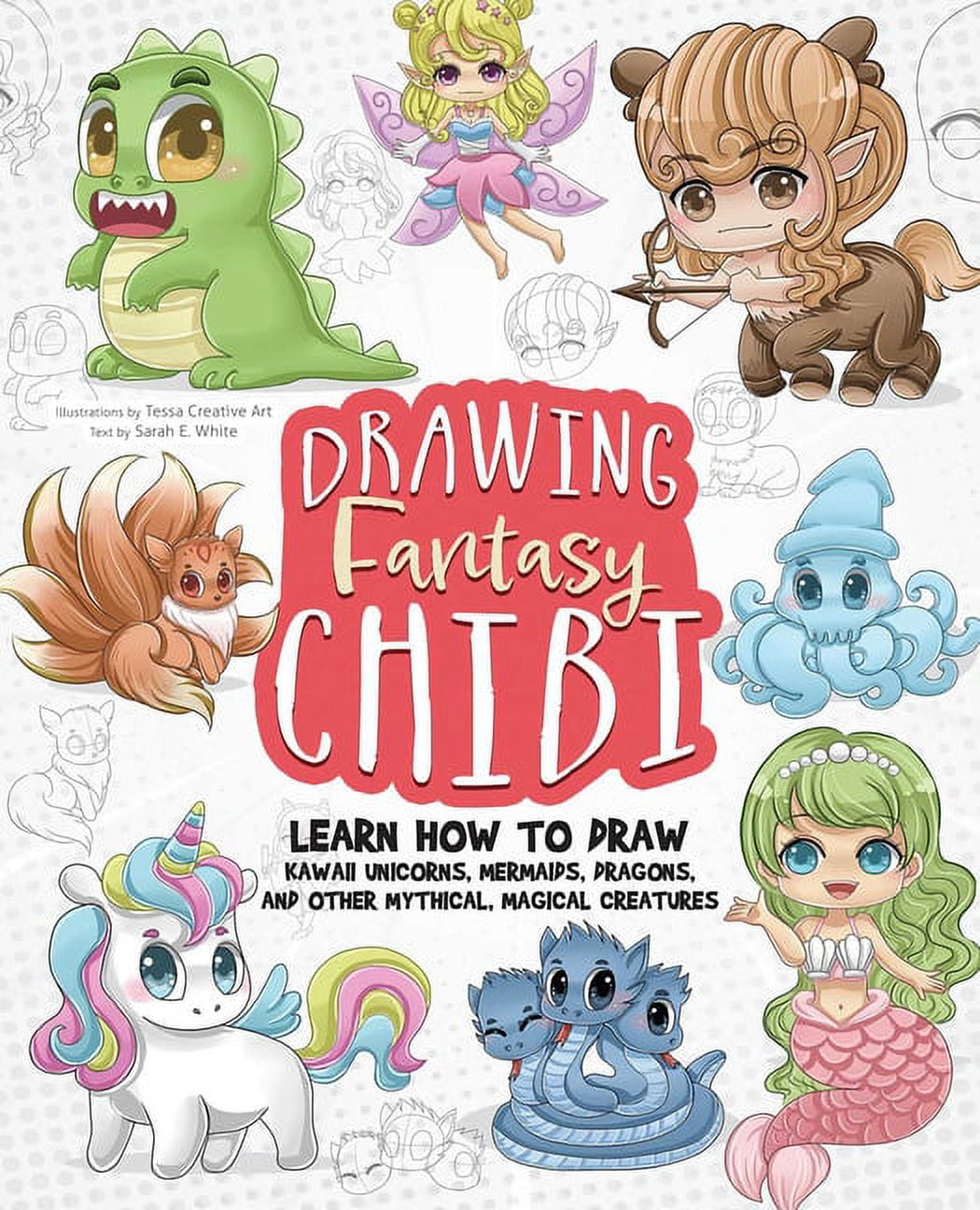This image is the cover of a how-to book titled "Drawing Fantasy Chibi." The title is prominently displayed in the center of the cover, with white text set against a dull red background. Beneath the title, in black text, the subtitle reads, "Learn how to draw kawaii unicorns, mermaids, dragons, and other mythical, magical creatures." Surrounding the text are eight illustrations of these fantastical characters, all rendered in a Japanese chibi style known for large eyes and disproportionately big heads. Featured illustrations include a green dinosaur in the top left, a magical pixie with purple wings in the top center, and a centaur with light brown hair holding a bow and arrow in the top right. The right edge also showcases a blue squid. The bottom row includes a mermaid with green hair and a pink tail, a unique interpretation of Medusa with red tongues, and a white unicorn with multicolored hair and blue eyes. Each colorized illustration is paired with a corresponding sketch to show the drawing process. The cover notes that illustrations are by Tessa Creative Art and text by Sarah E. White. This book is designed for those interested in learning how to draw these charming and whimsical characters.